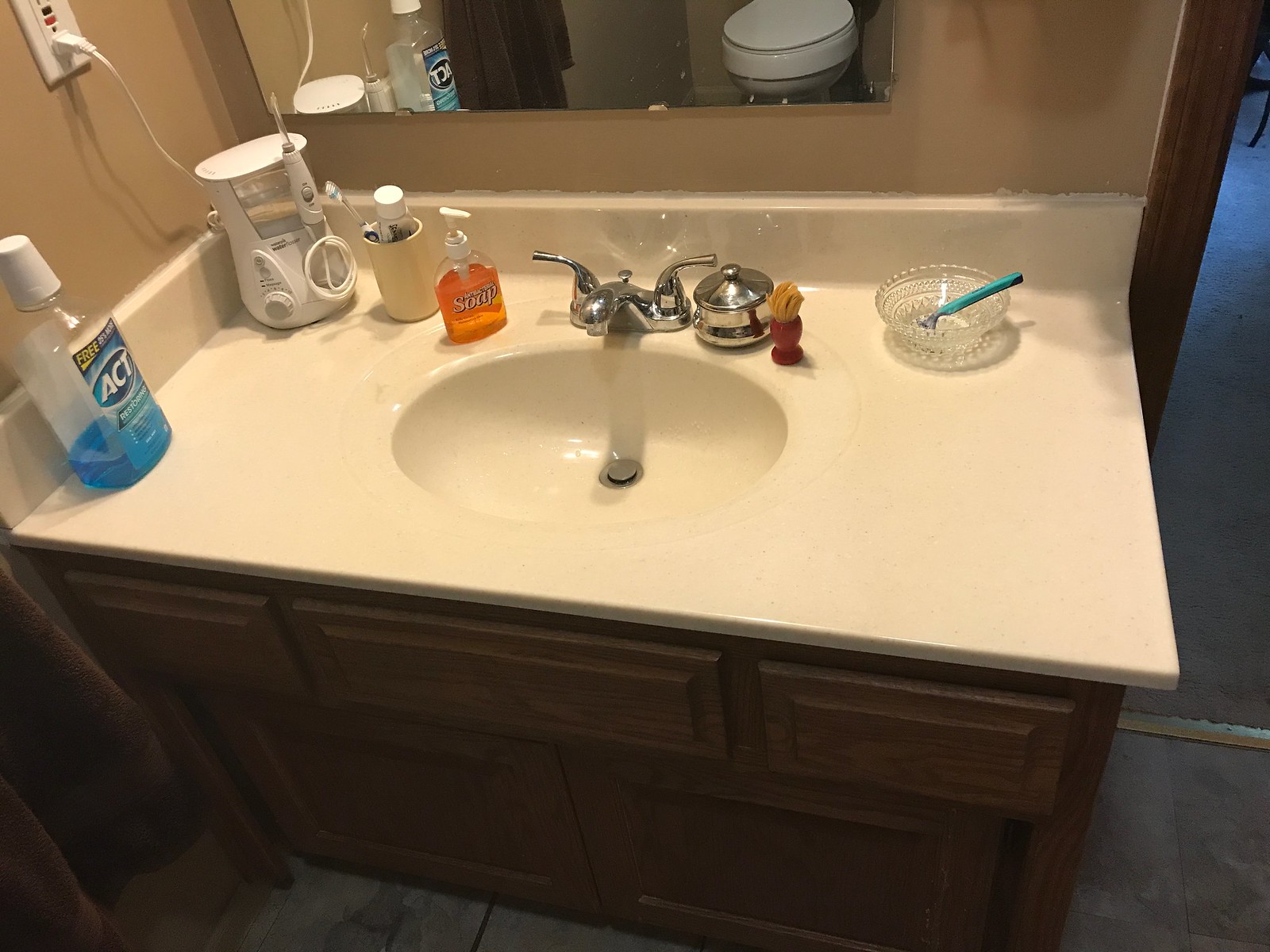The image features a bathroom sink area situated on a white countertop. Atop the countertop, there is a prominently displayed large bottle of nearly empty blue mouthwash with the label "ACT" visible on its surface. Accompanying it is a bottle of orange hand soap equipped with a white pump. A beige cup resides next to these items, holding a toothbrush and a tube of toothpaste. 

In the far left corner of the countertop, a small mechanical device, possibly a makeup brush, adds to the assortment of items. Additionally, a crystal-like bowl houses a blue razor.

Above the countertop hangs a mirror, providing a reflective surface, while the lower portion of the countertop is supported by wooden cabinetry. The cabinetry includes three drawers directly beneath the countertop, and two spacious cupboards for storage.

In the bottom left corner of the image, a glimpse of a brown shower curtain is visible, along with the beige-colored floor and walls. On the far right side of the image, part of a doorway is also in view.